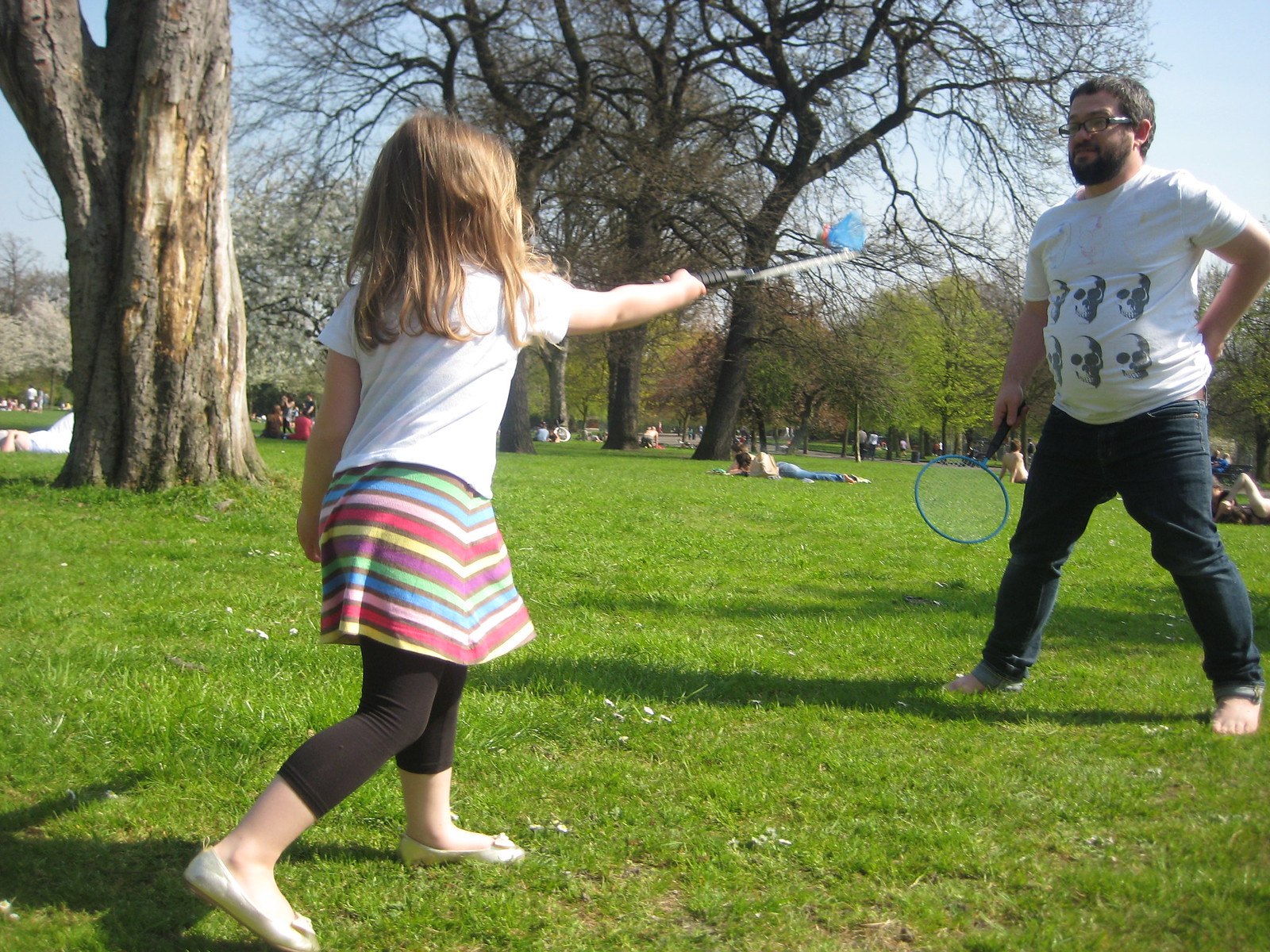In the photo taken outdoors, an older male and a young girl are engaged in playing a game in a park. The vibrant scene, though slightly blurry due to the action, captures the girl from the back dressed in a white shirt, a very colorful dress, and flats. In her hand, she appears to be holding something resembling a selfie stick, although it could also be a small, round badminton racket typically used in kids' games. The scene further includes a small triangular shuttlecock mid-air near the girl's racket. The older male stands close to the girl, participating in the game, and he is also holding a similar racket. The lush green grass and the presence of large trees, albeit with few leaves, set a serene background. The park is lively with other people—some are sitting, others lying on the grass, and a few walking in the distance. The sky is clear and sunny, enhancing the cheerful atmosphere of the day.